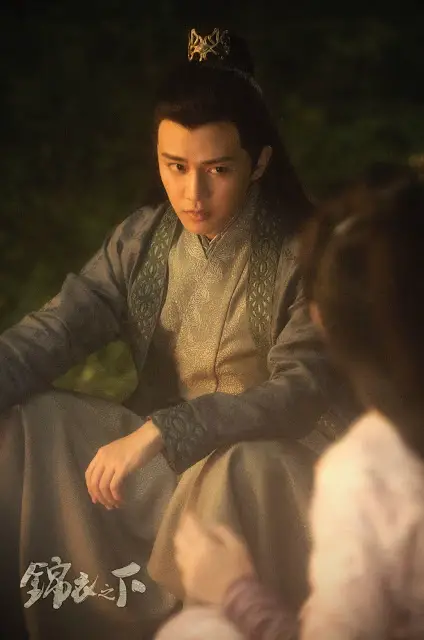The image is a color photograph, potentially a digitally created or artistically rendered poster or still shot from the TV series "Under the Power," featuring the actor Ren Julián. It shows Ren, dressed in traditional Asian ornamental attire, seated with one hand resting on his knee in a relaxed position. The background is an out-of-focus outdoor setting with hints of light greenery. Ren appears to be engaged in conversation with another person, whose face is not visible, only her shoulder and the back of her head seen in the bottom right corner of the image. The overall style is period costume with photographic representational realism. The image is in portrait orientation, featuring white-colored Asian text in brushstroke style on the lower left corner, adding an artistic touch to the composition.